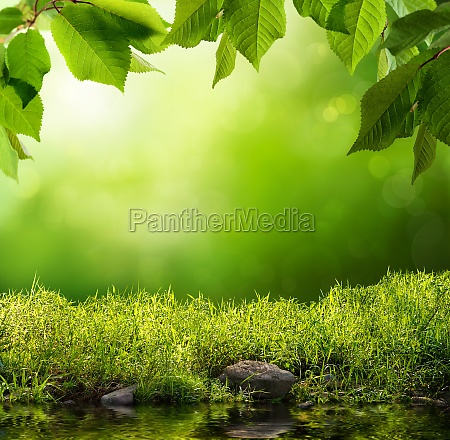The image is a computer-generated graphic design showcasing a lush, green marshland scene. At the bottom of the image, there is a tranquil pond with clear water, creating ripples that reflect the surrounding tall grass. The grass, which stretches from left to right, frames a medium-sized, square-like rock near the bottom center and a smaller rock slightly to the bottom left. The area above the water is adorned with dense, tall grass blades, contributing to the overall verdant landscape.

Further up, the image features a green, blurred background gradient that shifts from a dark green in the center and right to a lighter green towards the top left, where it suggests sunlight hitting the scene. Suspended from the top edge are green leaves, dangling and slightly obscuring parts of the image, adding a touch of nature's elegance. Among these leaves, small brown branches can be seen holding them in place.

Central to the image is an off-white watermark reading "Panther Media," somewhat transparent, allowing the greenery to be visible through the text. The dreamy, out-of-focus background along with the sharp details of the foliage and water make this scene an ideal choice for use as a serene and naturalistic background in various design projects.